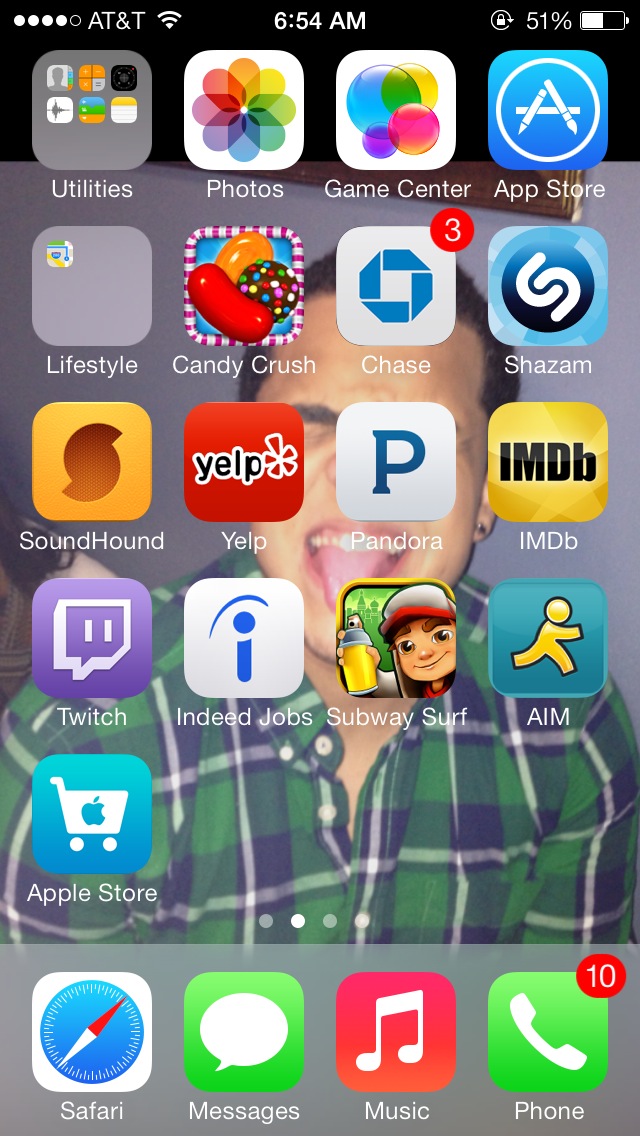This is a detailed screenshot of an AT&T cell phone, captured at 6:54 AM with a battery charge of 51%. The display shows various apps neatly organized in four rows of four icons each, followed by a final row containing only the Apple Store icon. Among the visible apps are Utilities, Photos, Game Center, App Store, Lifestyle, Candy Crush, Chase, Shazam, SoundHound, Yelp, Pandora, IMDB, Twitch, Indeed Jobs, Subway Surf, AIM, and the Apple Store. At the bottom of the screen, there are the essential apps: Safari, Messages, Music, and Phone. Above the Phone app icon, there is a red notification badge indicating 10 calls or voicemails. The background image features a man wearing a blue, green, and white plaid shirt with an open neck, sticking out his tongue and closing his eyes in a humorous expression.